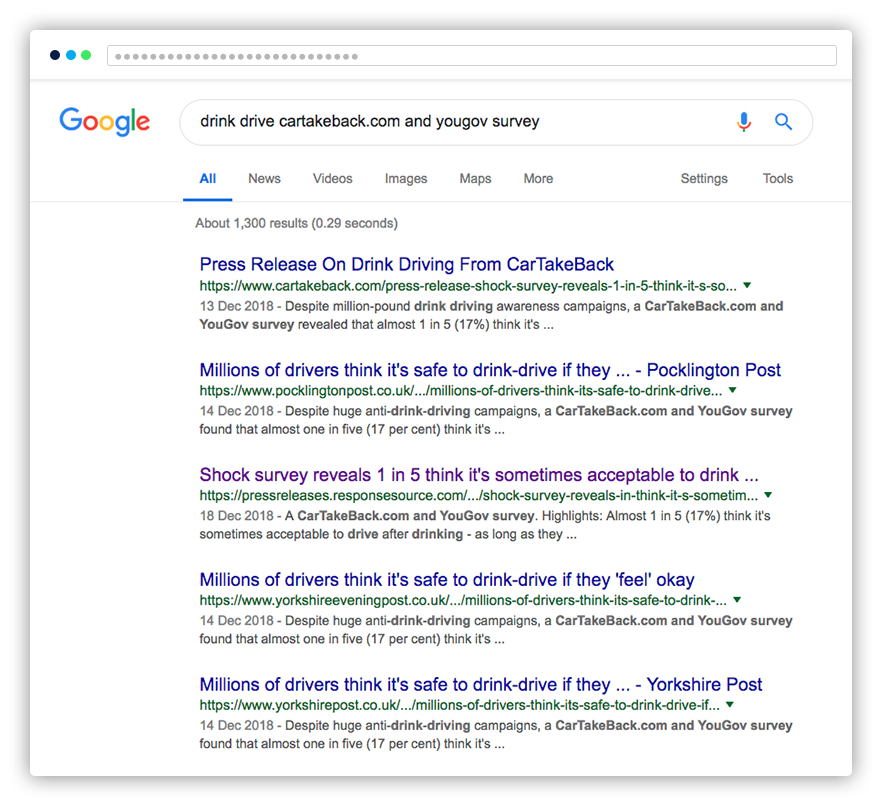This image is a detailed screenshot taken in landscape mode of the Google website interface. It features several distinct elements:

1. **Upper Left Corner**:
   - Three dots: one black, one blue, and one light green.

2. **Central Portion**:
   - A large rectangle containing twenty-eight small gray dots arranged in a grid pattern.

3. **Main Content**:
   - The Google logo is prominently displayed beneath the dot grid.
   - In the search bar, the query reads, "drink drive car take back.com and you go survey." To the right of the search bar, there are the microphone icon and search icon.

4. **Navigation Tabs**:
   - Active tab underlined in blue: "All."
   - Other available tabs include "News," "Videos," "Images," "Maps," "More," "Settings," and "Tools."

5. **Search Results**:
   - Displays approximately 1,300 results, retrieved in 0.29 seconds.
   - The first five search result links are detailed:
     1. **First link (in blue)**: "Press release on drink driving from car take back."
     2. **Second link (in blue)**: "Millions of drivers think it's safe to drink drive if they" (from Pop Wington Post).
     3. **Third link (in purple)**: "Shock survey reveals one in five thinks it's sometimes acceptable to drink" (visited link).
     4. **Fourth link (in blue)**: "Millions of drivers think it's safe to drink drive if they feel okay."
     5. **Fifth link (in blue)**: "Millions of drivers think it's safe to drink drive if they" (from Yorkshire Post).

This thorough description provides a comprehensive overview of the Google search interface and the specific search query results.